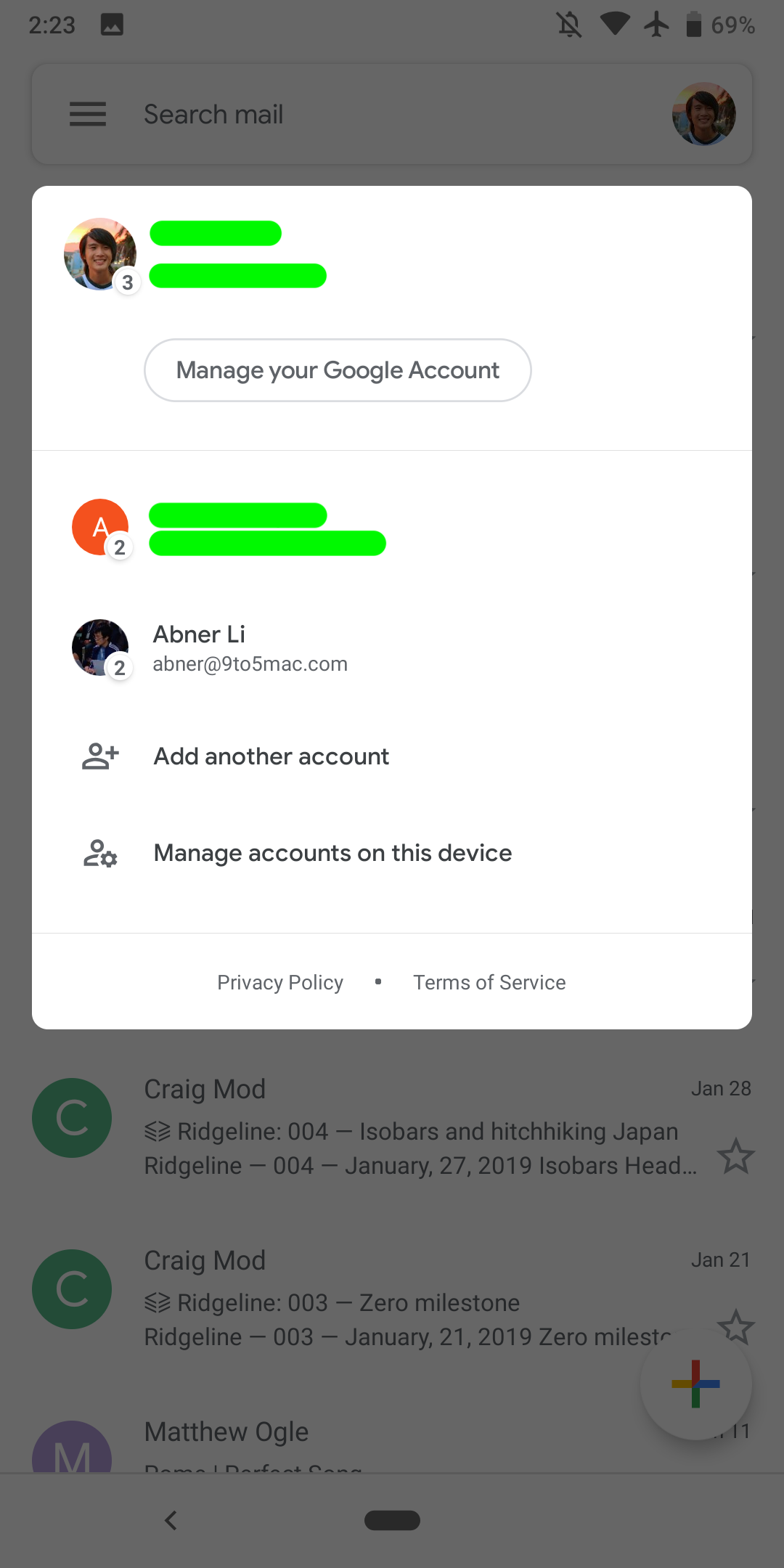**Screenshot Description:**

The screenshot showcases a mobile device screen primarily focused on a white pop-up with rounded corners that overlays the dimmed main content. At the very top, the mobile UI icons are visible: on the left, the time "2:23 PM" in dark letters, and an image icon indicating a screenshot. On the right side, several icons are displayed: a notifications-disabled icon, a fully connected Wi-Fi icon, an airplane mode icon, and a vertical battery icon with "69%" next to it.

Below these icons lies the Gmail interface, indicated by a "search mail" bar with the user's profile picture—an image of an Asian male with black hair in an outdoor setting. Below this bar, the white pop-up begins. Various user actions have masked some information for privacy, marked by green edits. The pop-up shows:

1. An avatar with the number "3" inside, followed by two green lines covering sensitive information.
2. The text "Manage your Google account."
3. Another avatar, a white "A" on an orange background with the number "2" inside, again partially obscured by green lines.
4. A third avatar with the number "2" inside, showing the name "Abner Lee" and an email address starting with "abner" followed by indistinct digits and a partial domain.

Additional options in the pop-up include "Add another account," "Manage accounts on this device," "Privacy Policy," and "Terms of Service."

In the dimmed background behind the pop-up, partially visible Gmail content from the user's inbox can be seen. Three rows include:

1. An entry from Craig Maude with a green circle and white icon, mentioning "Ridgeline 004, Isobars, and Hitchhiking Japan," alongside dates "Ridgeline 004, January 27, 2019" and "Isobars, January 28."
2. Another entry, partially visible from Matthew Ogle.

The screenshot's frame ends just above the mobile device's navigation bar, which includes: a centered oval representing the home button, a left-facing arrow symbol ("<") on the left side, and a circular icon with a "+" sign on the right, presumably to compose a new email.